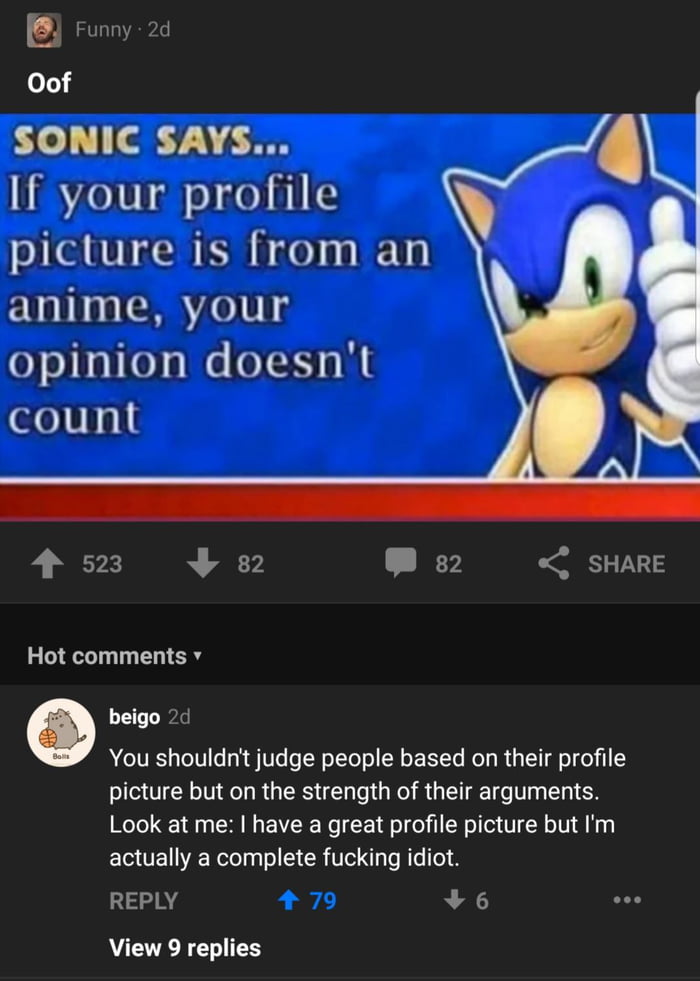In the image, we observe what appears to be a meme at the top left, featuring a square box with a laughing person's face. The individual has a light skin tone, a dark beard, and is looking upward as they laugh. To the right of this box, the word "funny" is visible, accompanied by "2D," indicating the meme is two days old. Below this, the word "oof" is displayed in white text.

The central section of the image showcases another squared box with text at the top left that reads, "Sonic says..." followed by, "if your profile picture is from an anime, your opinion doesn't count." To the right of this text is an image of Sonic the Hedgehog giving a thumbs-up. Sonic is characterized by his blue fur, light brown belly, arms, and inner ears, green eyes, a black nose, and white gloves.

Beneath this section are icons for thumbs up, thumbs down, comment, and share. The thumbs up icon shows a count of 523, the thumbs down icon shows a count of 82, and the comment icon also shows a count of 82.

At the very bottom of the image, the section labeled "hot comments" features a remark from a user named Bjo, who states, "You shouldn't judge people based on their profile picture, but on the strength of their arguments."